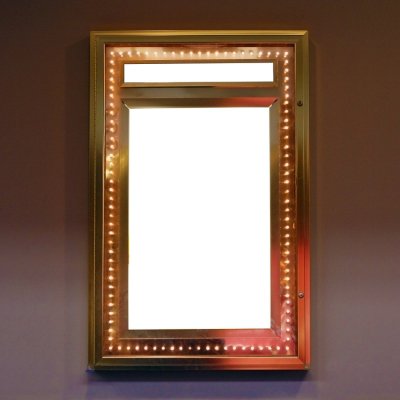This image features a 3D graphic art depiction of a mirror or picture frame set against an ombre background that transitions from a dark maroon at the top to a lavender hue at the bottom. The centerpiece of the image is a gold-framed structure possibly resembling a mirror or a poster display. The frame itself has two distinct textures: the outer edge is a smooth solid gold, whereas the inner edge features a tarnished gold with symmetrical rivet-like bumps. The interior of the frame is primarily white, with a horizontal gold strip adorning the top. Encircling the entire frame, yellow dots or lights are embedded within the brown to reddish background. This detailed visual setup suggests an artistic portrayal of an ornate, illuminated display, potentially akin to a movie poster lightbox or a decorative mirror.